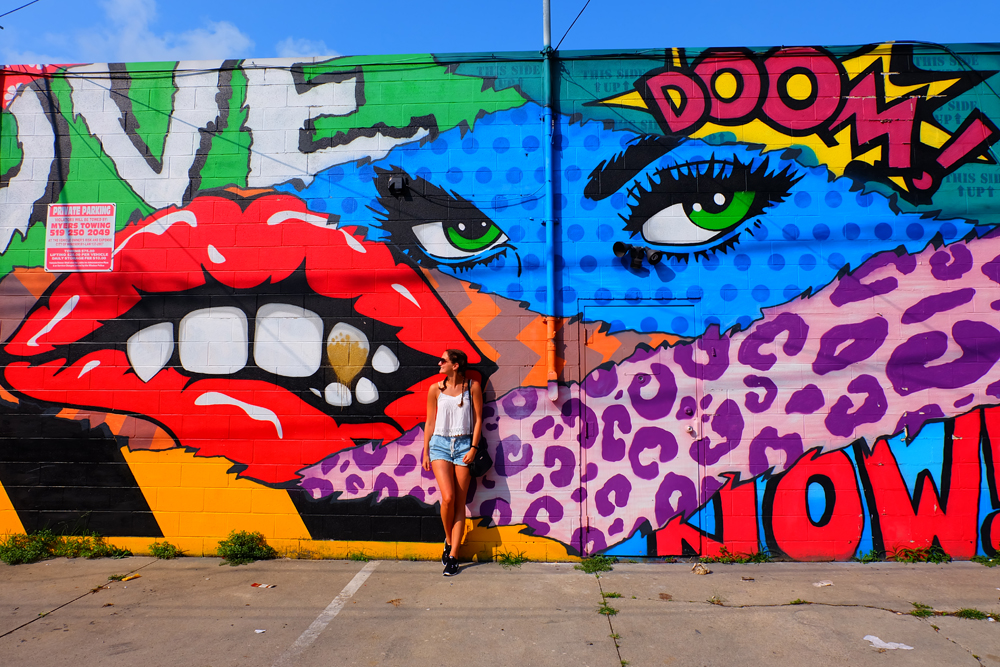A vibrant photograph captures a young woman with brown hair styled in pigtails standing in front of an elaborate and colorful graffiti art wall on what appears to be a parking lot. The ground is marked with parking spaces and some weeds growing through the cracks. The wall, possibly the side of a building, is adorned with a myriad of comic book-style elements and bold colors. Prominently displayed in large red lettering is the word "DOOM" with a yellow lightning bolt on a green background. Below this, a pair of intense green eyes stare out from a blue polka dot background, accentuated by heavy eyebrows and eyelashes. There is also a striking pair of vampire-like lips biting down, beneath which are orange and black zigzag patterns. Additional graffiti includes words such as "NOW" in red comic book-style lettering on a blue background, and an area that spells out "LOVE" partially visible with the letters O-V-E. Another section features pink and purple cheetah print motifs. The woman, dressed in short blue jean shorts, a white tank top, black tennis shoes, and sunglasses, poses facing to her right with one leg bent and her arms relaxed at her side, completing this vivid urban tableau.